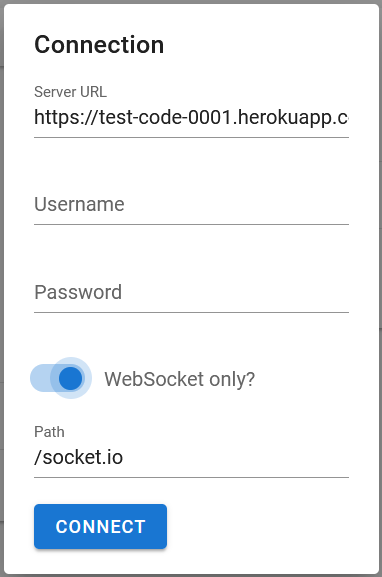The image features the layout of a connection configuration interface within a vertically aligned rectangle.

1. **Outline and Title**: The rectangle is bordered in gray, with the heading "Connection" at the top.
2. **Server URL**: Directly beneath this is the label "Server URL" in uppercase. Below this label is a URL: `https://test-code-0001.herokuapp.com`.
3. **Username and Password Fields**: The image displays two input fields:
   - **Username**: Marked by a label "Username" with a long horizontal line below it.
   - **Password**: Marked similarly by the label "Password" with its respective long horizontal line.
4. **WebSocket Toggle**: Following these fields is a toggle switch area. The circular toggle, colored dark blue, is positioned to the right, indicating the active state. Beside this toggle, the text "WebSocket only?" appears in gray.
5. **Path**: Below the toggle area, the text "Path" is shown, followed by a dash and the path `socket.io`, with "socket" spelled as "S-O-C-K-E-T".
6. **Connect Button**: At the bottom of the rectangle, a solid blue rectangle prominently displays the word "CONNECT" in all uppercase letters and white font.

This detailed description provides a comprehensive overview of the interface elements and their arrangements within the image.